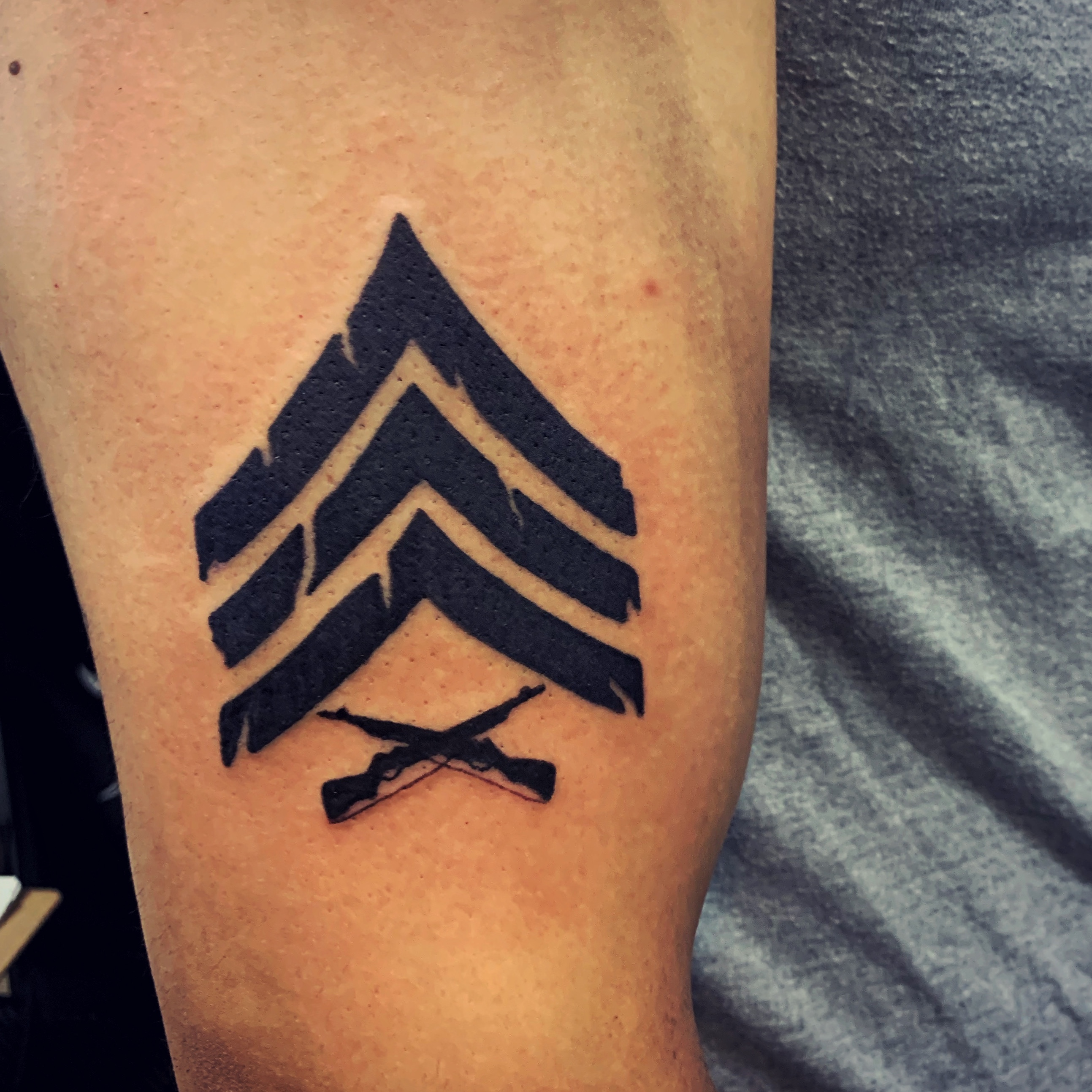This is a detailed close-up photograph showcasing a fresh tattoo on a man's left arm. The tattoo features a military-inspired design consisting of three inverted V-shapes with jagged edges and cracks, positioned above two rifles that are crossed in an X pattern. The tattoo appears recent as the skin around it shows signs of redness and irritation. The image captures the arm clearly, emphasizing the bicep and tricep muscles, with the backdrop being a gray fabric, likely the man's tank top shirt. Additionally, a small mole is visible on the upper left-hand corner of the arm, adding a natural detail to the visual.